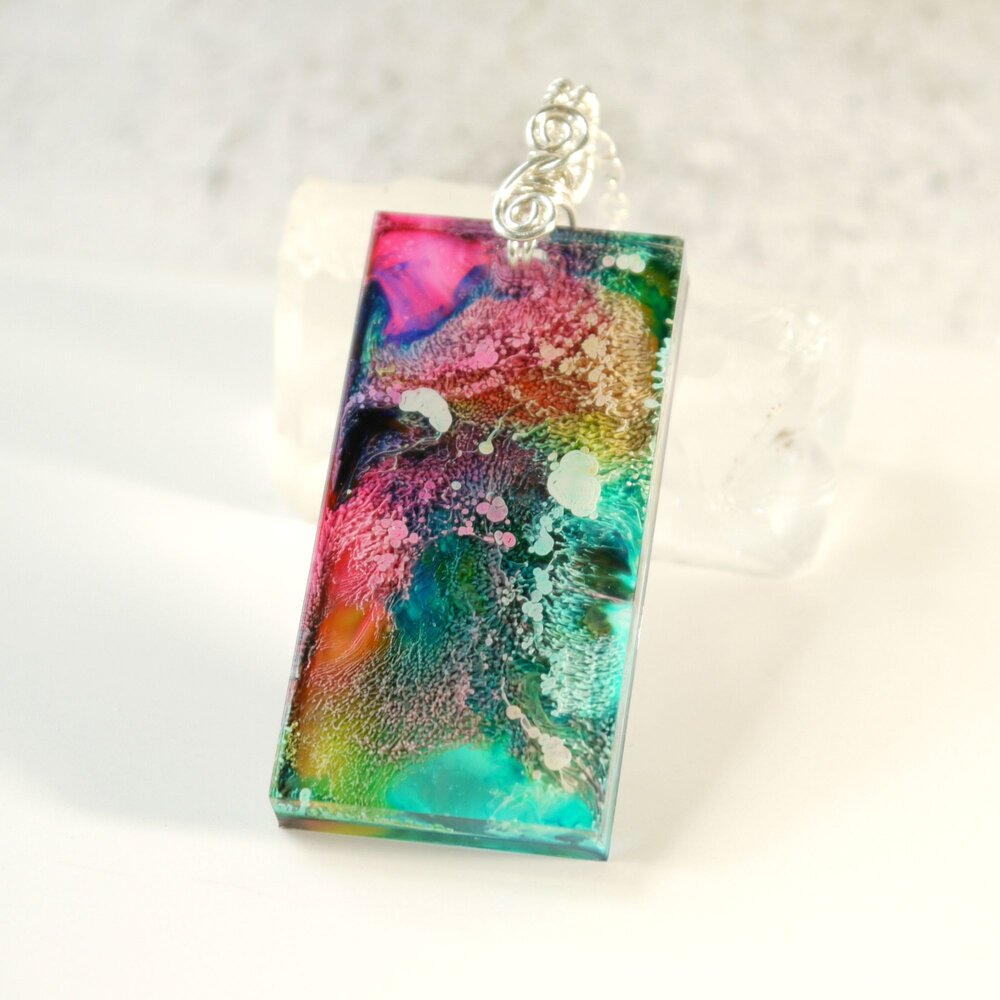This image captures a close-up photograph of a striking and artistic piece of jewelry—a pendant designed to resemble a rectangular bar, which is vertically oriented. The pendant features a vibrant mix of colors reminiscent of an abstract painting, with splashes and blotches of blue, red, purple, turquoise, and hints of orange, creating a unique, textured appearance. The pendant appears to be made from a material resembling beveled glass or resin, giving it a polished and dynamic look. At the top of the piece is a delicate metallic clasp, likely made of either white gold or silver, designed to attach to a silver chain necklace, although it could also function as a brooch. The colorful pendant is set against a plain, beige background, which highlights the pendant's vivid colors and intricate details, making it the focal point of the image.